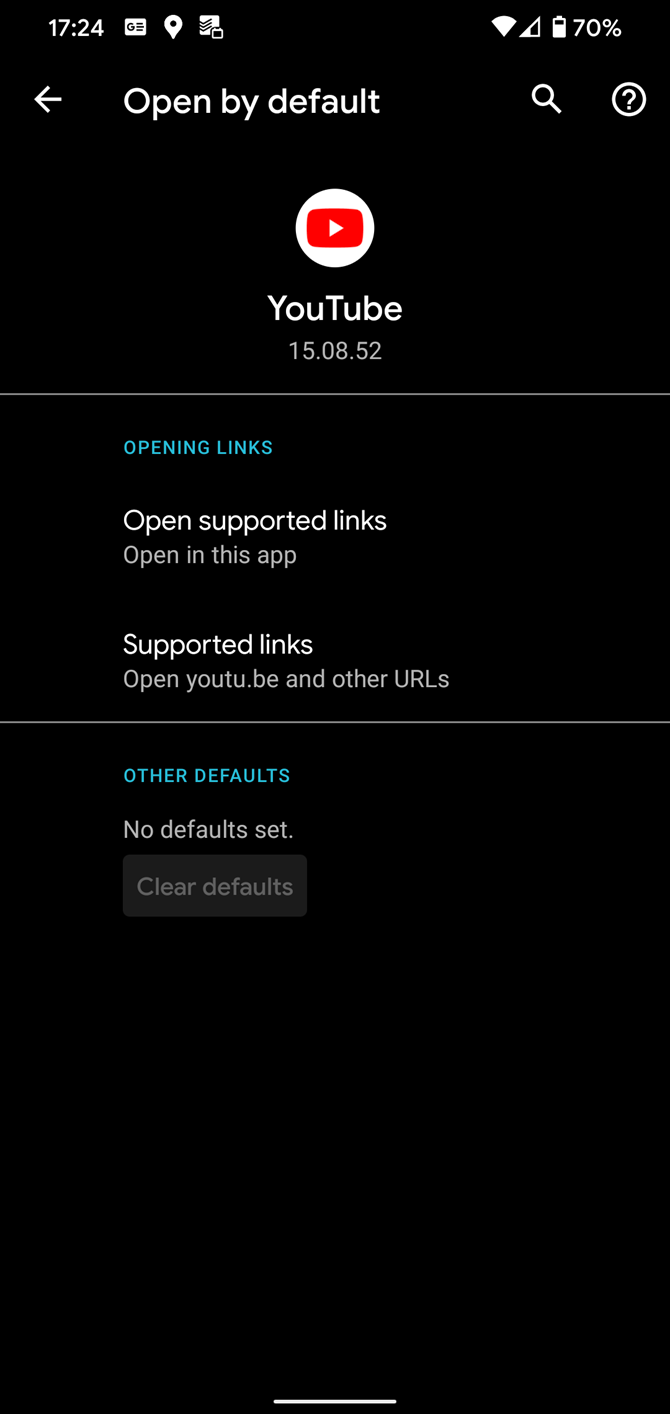This image is a detailed screenshot from a smartphone displaying a settings menu on a pitch-black background. 

At the top-left corner, the time is shown in white font as "17:24," indicating the 24-hour clock format. On the top-right, there are several icons: the battery icon, indicating a 70% charge, the WiFi icon, and the wireless connection icon.

Below these system indicators, a headline in bold white font reads "Open by default," accompanied by a white left-pointing arrow adjacent to it. Centrally located beneath the headline is the YouTube logo, consisting of a red square with rounded corners containing a right-pointing triangle, all encircled by a white circle. Beneath this logo, the word "YouTube" is written in white font, with "15.08.52" displayed below in gray font.

A very thin gray line separates this section from the next, where the text "Opening links" is displayed in blue font. Below this, the white text "Open supported links" appears with the gray text "Open in this app" underneath. Following this, "Supported links" is written in white font with "Opening YouTube and other URLs" in gray beneath it.

Another thin gray line demarcates the next section, which reads "Other defaults" in blue font, followed by "No defaults set" in gray font. The screenshot is concluded with a very dark gray rectangle at the bottom, contrasting slightly against the black background, containing the text "Clear defaults" in gray font.